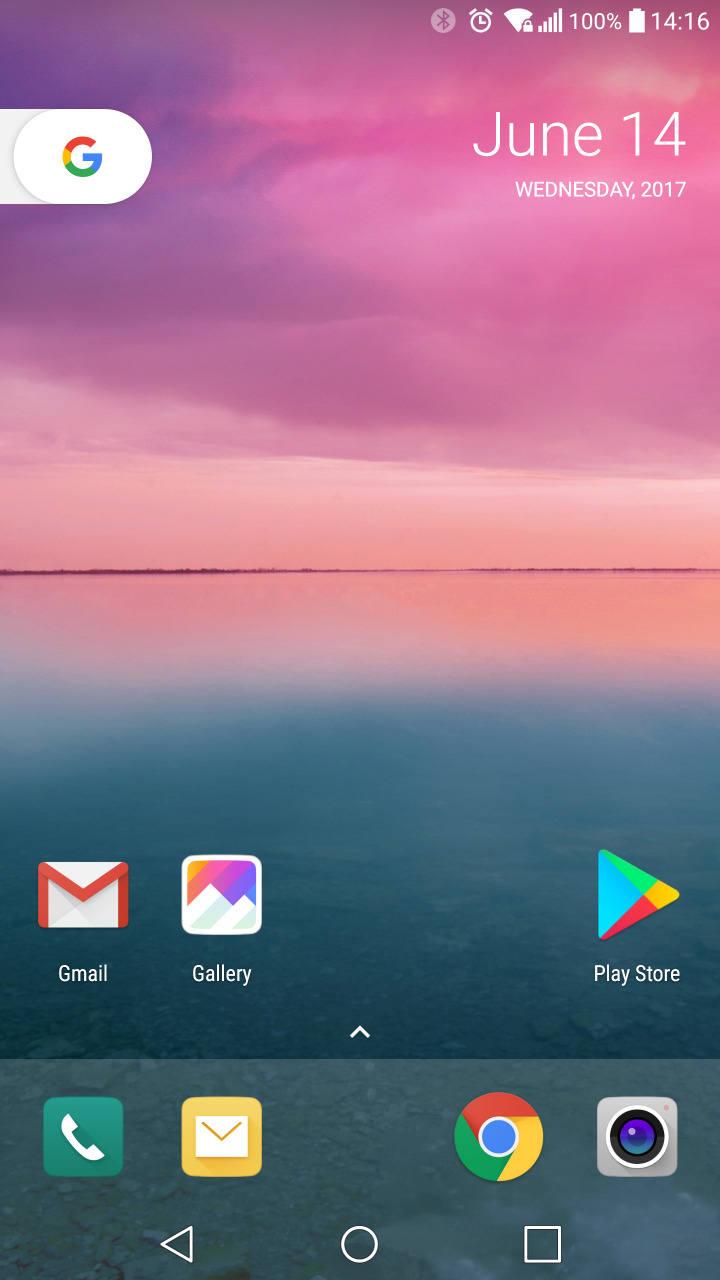A detailed cellphone home screen screenshot features a serene background image composed of a tranquil water surface at the bottom. Midway through the image, a dark horizontal line separates the water from the sky, which transitions into a peach color gradient that further evolves into a vibrant, cloudy mix of purple, pink, and orange hues at the top.

The top-right corner displays essential phone icons in white. Approximately five lines down from the top, on the left side, half of a gray oval emerges, featuring a white oval on its right side, housing Google's multicolored "G."

On the far right side, "June 14" is prominently displayed in white text, below which "Wednesday, 2017" is written.

The bottom part of the screen consists of two rows of app icons. In the top row, starting from the left, are the Gmail icon and the Gallery icon, followed by two blank spaces, and ending with the Play Store icon. Centered below is a white, upward-pointing arrow, resembling an upside-down "V." The bottom row contains icons for Phone and Mail on the left, a blank space in the middle, and the Chrome and Camera icons on the right. There is no text beneath these icons.